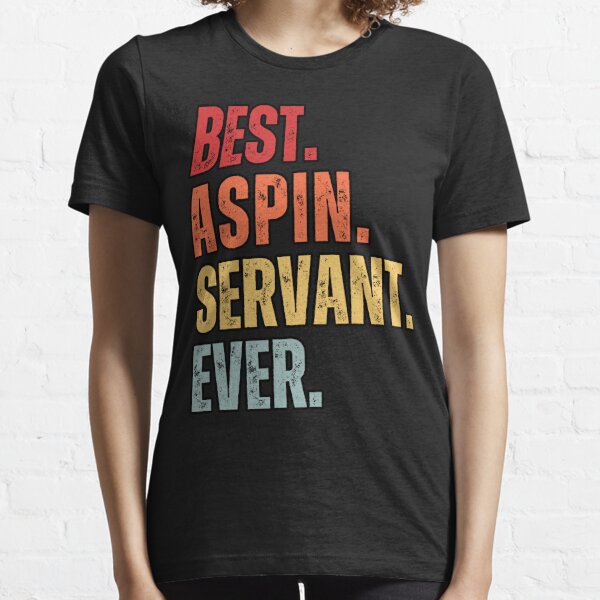The image shows a white woman with some visible brown hair, modeling a black short-sleeved t-shirt. Her arms are hanging down, and although her face is not visible, you can see her neck. The t-shirt has four lines of text, each uniquely colored: "BEST." is in red, "ASPEN." is in orange, "SERVANT" is in yellow followed by a yellow dot, and "EVER" is in blue with a blue dot. The background features a white brick wall, providing a clean, simple backdrop. The overall impression is one of casual fashion with a playful use of color in the text.